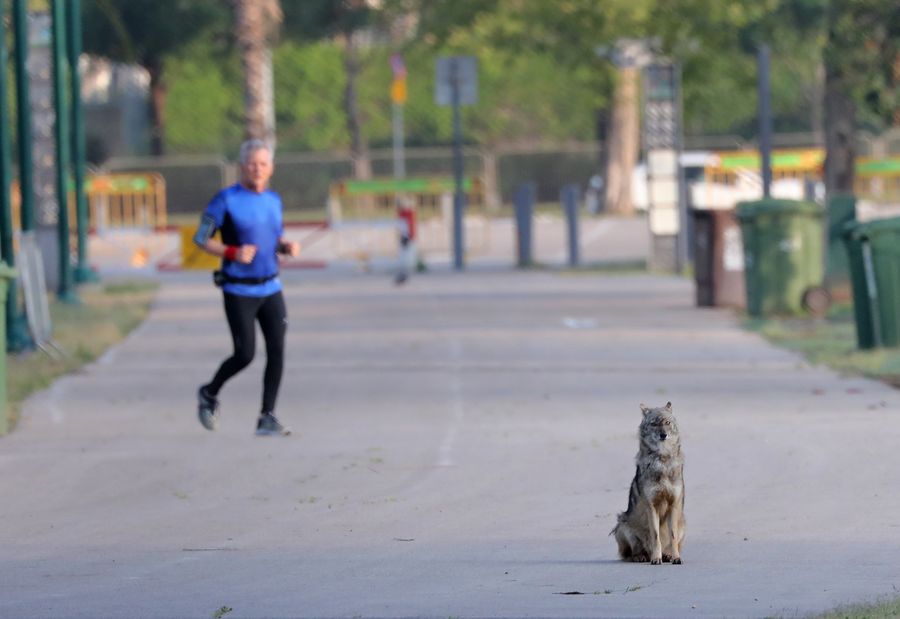In this horizontally aligned rectangular photograph, the main focus is on a small grayish-brown coyote sitting erect in the middle of what seems to be the entrance to an older parking lot. The coyote, with its short pointed ears, is staring directly at the camera. Behind it, slightly to the left, is a blurry image of a surprised older white man with white hair, dressed in black leggings, running shoes, and a tight-fitted blue shirt with a red armband. He appears to be jogging but has paused and is also looking towards the camera. Surrounding elements include green trash and recycling bins on the right, gray street signs, and gates marking the entrance to the parking lot, adding to the environment of an urban park or lot. The overall atmosphere is one of a curious and unexpected encounter captured on a blurry but interesting photograph.